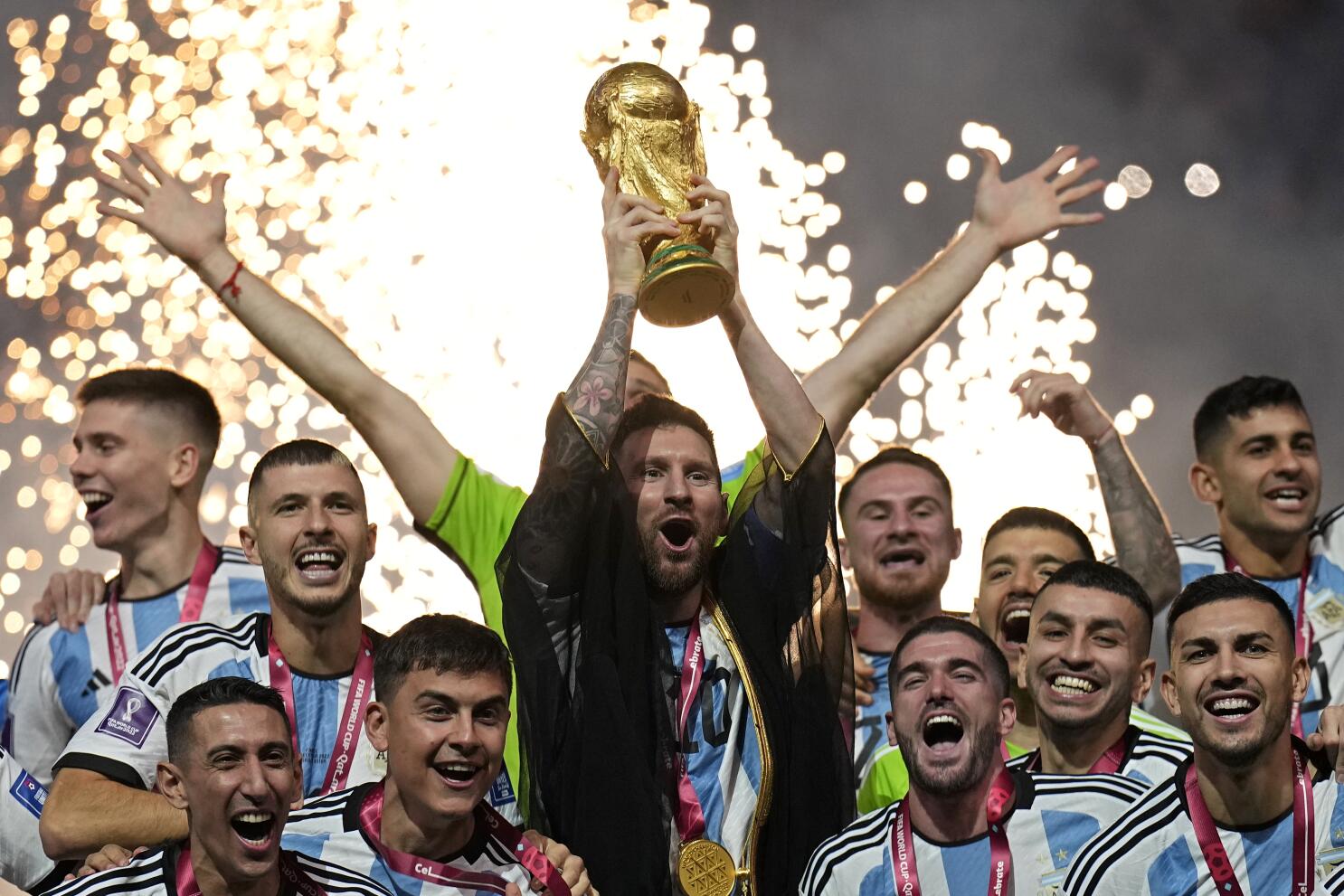In this image, a triumphant celebration is taking place at nighttime or late evening, captured in a rectangular, landscape-oriented photograph. Centered in the image is a man, elevated above the rest, who is holding a golden trophy topped with a ball. He is adorned in a sheer black robe over a blue and white striped uniform. Around his neck, a red lanyard can be seen, likely sporting the inscription "FIFA World Cup" and possibly "Qatar". His left arm, which features a prominent tattoo, hugs the trophy as he grins joyfully.

Surrounding him is a group of men, all donning identical blue and white uniforms reminiscent of the Argentina soccer team's kit, each also wearing red lanyards. Their expressions are exuberant, their mouths open in mid-cheer, and their hands raised in excitement. Behind the man holding the trophy stands another individual in a green shirt, arms outstretched, seemingly part of the jubilant scene.

Illuminating the background are dazzling white and gold fireworks, casting a brilliant light over the joyful scene, while gray smoke wafts through the air, adding to the celebratory atmosphere. The photograph captures the elation and unity of the team as they revel in their hard-earned victory.